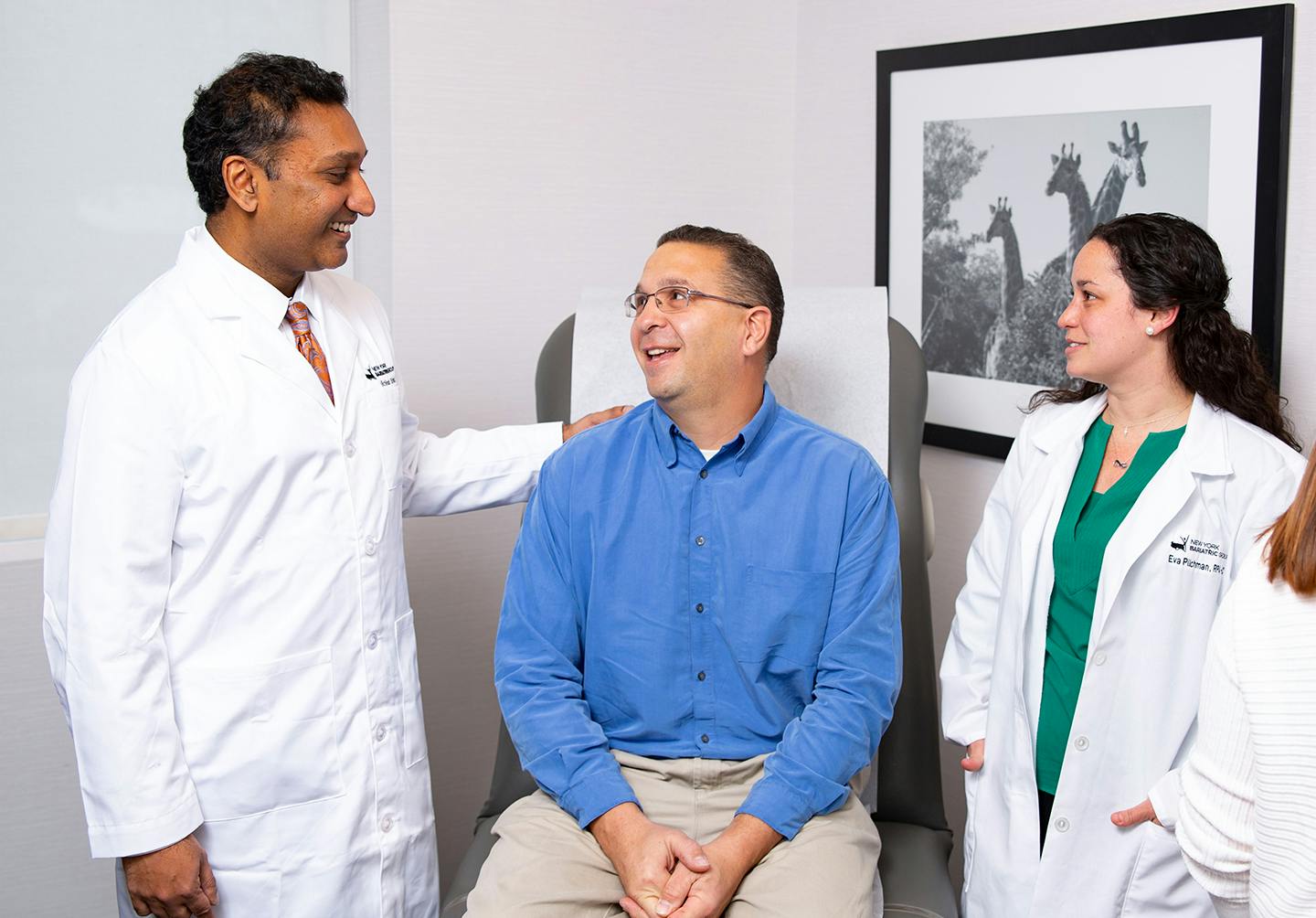In this detailed image of a doctor's office, three main figures are captured. At the center, an older gentleman, likely in his 40s or 50s, is seated on a gray doctor's chair with white paper covering. He is wearing a blue button-up shirt, khaki pants, and glasses, and he has his hands resting in his lap while smiling warmly. To his left, a male doctor with gray hair, dressed in a white coat over a red tie, is smiling and looking directly into the patient's eyes. The doctor's coat features black text indicating his name and practice, although the specific details are indiscernible. The doctor's hand rests reassuringly on the patient's shoulder. On the man's right side, and the picture's left side, stands a female doctor or nurse, identifiable by her long black hair and green shirt beneath her white coat. She is also smiling as she looks at the patient, with her hands possibly in her pockets. Behind this trio, a white wall serves as a backdrop, adorned with a black-framed image of three gray-toned giraffes among trees. A fourth character, whose face is not visible but has reddish hair and appears to be wearing a white sweater, is partially seen on the far right side of the image.